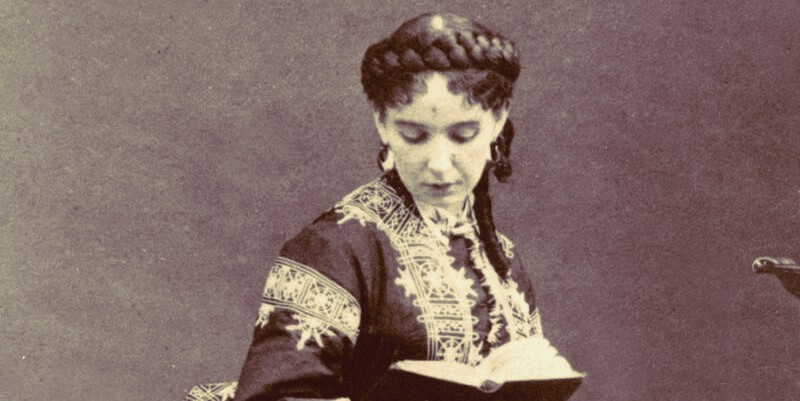This black and white photograph features a woman with dark hair intricately braided into a thick, horizontal plait running across the top of her head. She gazes downward towards an open book held in her right hand, the book itself about three-quarters open with visible white pages and a dark cover. The backdrop of the image is a dark, plain background that further accentuates her detailed attire and accessories. The woman is clad in an ornate robe characterized by fanciful sun embroidery that extends down the front in a stole-like pattern and decorates the upper sleeves. Her elaborate outfit resembles a fitted jacket over a dress, adorned with intricate, gold-like trimmings. Notably, she has a small jewel on her forehead and dangles earrings, adding to her elegant and possibly priestess-like appearance. The photograph captures her from head to chest, highlighting the exquisite details of her garment and her downward-focused, contemplative expression.